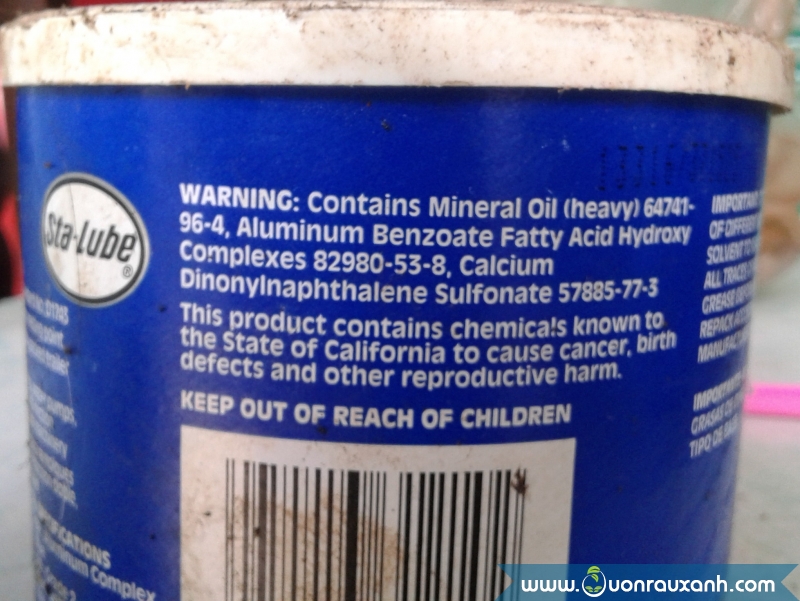This image is a close-up of a cylindrical container slightly wider than it is tall, likely used in a garage setting due to its dirty appearance. The container has a white, snap-on plastic lid that appears very grimy. The main body of the container is medium blue. On the left side of the label, there is a logo that reads "STA-Lube" in black lettering within a white background and encircled by a black perimeter. The core of the image is dominated by white text that serves as a warning label. It details the contents such as mineral oil (heavy, CAS number 64741-96-4), aluminum benzoate fatty acid hydroxy complexes (CAS number 82980-53-8), and calcium dinonylmethyl sulfonate (CAS number 57885-77-3). Additionally, the label warns that the product contains chemicals known to the state of California to cause cancer, birth defects, and other reproductive harm, advising to keep it out of reach of children. The container sits on a white surface with a blurry background, indicating age and heavy use. In the lower right corner, there is a stylized watermark reading "www.unrauxanh.com."